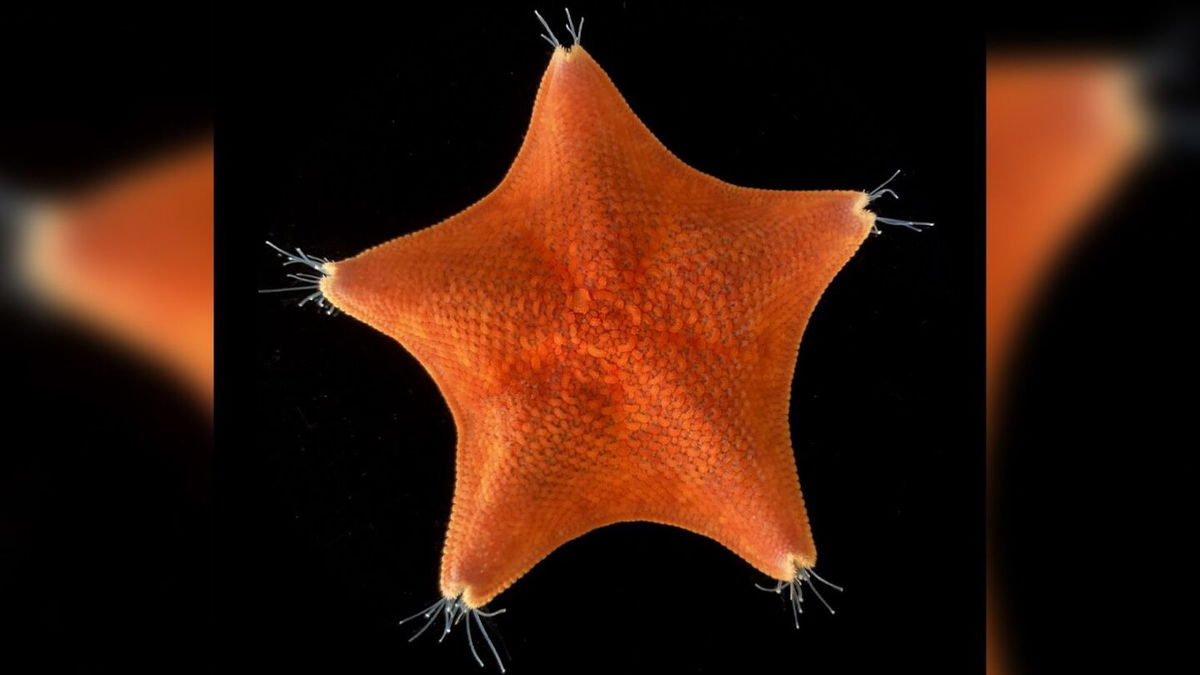A striking close-up photograph captures a vibrant, live Galabraster Antarctica red spiny cushion starfish, positioned against a deep black background that enhances its vivid burnt orange hue and amber-tipped extremities. The starfish, showcased in a rectangular frame, appears with its five arms prominently extending from a central hub, where visible vein-like structures branch out towards each arm's tip. Each point of the starfish bristles with fine, hair-like tendrils, resembling tiny whiskers emerging from its rough, textured surface. The image reveals intricate details such as the starfish's scales and indentations, emphasizing its dynamic and lively nature. Additionally, blurred, shadowy extensions of the starfish on the left and right sides suggest a transposed shadow, adding depth and focus to the central bright starfish, making it stand out vividly against the dark backdrop.